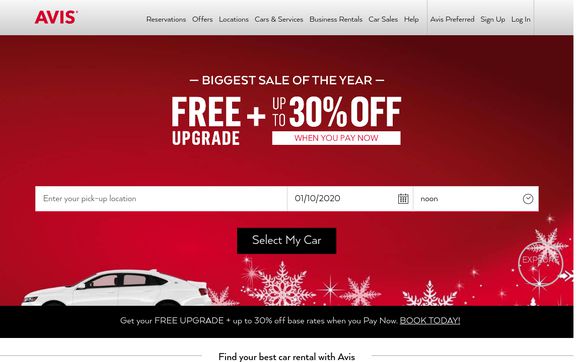This image showcases the Avis website. At the top, there is a light gray banner featuring "Avis" in bold red, capitalized text. The navigation menu includes the following options: Reservations, Offers, Locations, Cars & Services, Business Rentals, Car Sales, and Help. Additionally, there are links for "Avis Preferred Sign Up" and "Log In."

Below the banner, a red background gradient appears, deepening at the corners. In the center of this background, the text "Biggest Sale of the Year" is displayed prominently. Underneath, in larger and bolder font, it states "Free Upgrade Plus Up to 30% Off." A white band below this contains the text "When You Pay Now," highlighted in red font.

Further down, a white search bar allows users to enter their pickup location. The placeholder text includes a date "01/10/2020" and the time set to "Noon." Below this is a black banner with white text that reads "Select My Car."

To the left, there is an image of a white car, complemented by snowflake and ornament graphics, suggesting a holiday theme. Another black banner at the bottom encourages users with the message: "Get Your Free Upgrade Up to 30% Off Base Rates When You Pay Now. Book Today."

Finally, outside of this graphic, a call-to-action at the bottom of the image reads, "Find Your Best Car Rental with Avis."